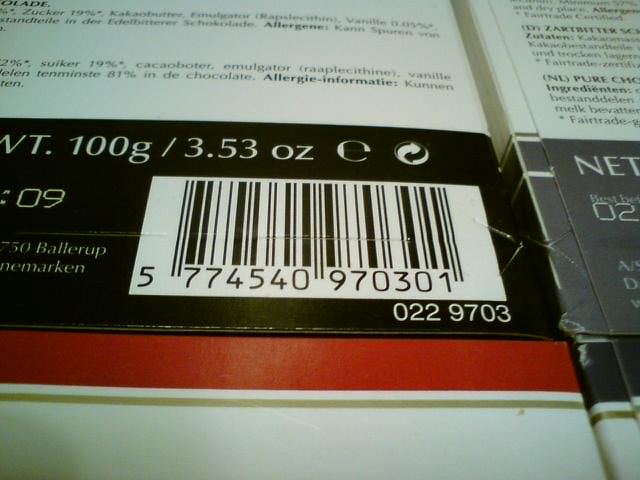A close-up image revealing the UPC code on the back of a white box with black and red accents. The box specifies a weight of "WT. 100 grams / 3.53 ounces." Prominently displayed, the UPC code reads "5774540970301," with additional identification numbers "0229703" situated right below. The background also shows sections dedicated to ingredients and allergy information, hinting at the product's content and dietary considerations.